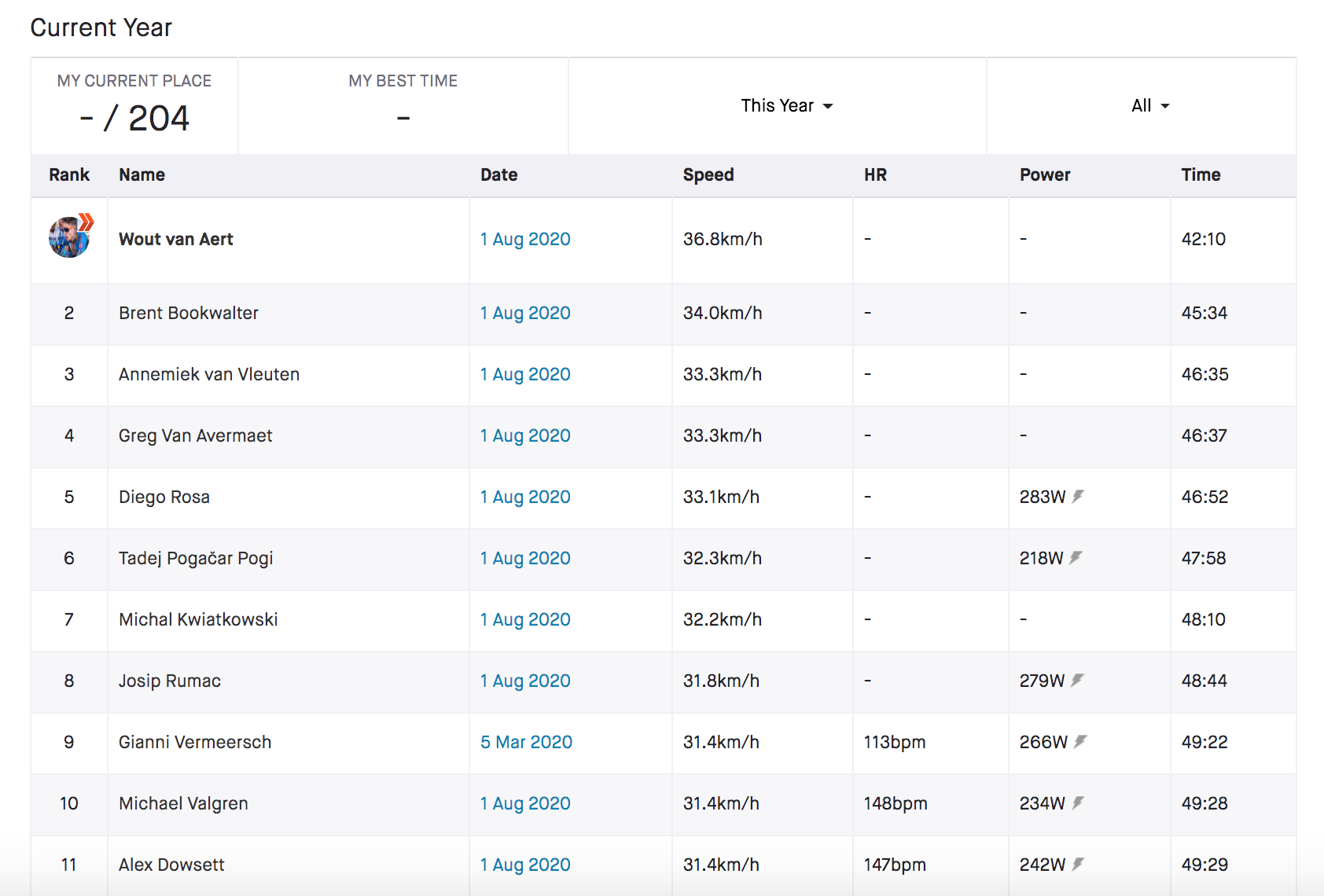This page features a detailed table against a white background. In the upper left corner, it reads "Current Year". Below this heading, the text "My Current Place - 204" is displayed. To the right, another text block shows "My Best Time -", followed by two labeled boxes: "This Year" and "All".

Dominating the page is a well-organized table, which is segmented into columns labeled as: Rank, Name, Date, Speed, HR (heart rate), Power, and Time. The names listed in the table, arranged by rank, include:

1. Woot Van Aert
2. Brent Bookwalter
3. Annemiek van Vleuten
4. Greg Van Avermaet
5. Diego Rosa
6. Tadej Pogačar
7. Michał Kwiatkowski
8. Joseph Rummik
9. Gian Ramesh
10. Michael Valgren
11. Alex Dowsett

The "Date" column features green text with left-pointing arrows, indicating a uniform date for all entries: August 2020.

In the "Speed" column, the recorded speeds are:
- 36.8 km/h
- 34 km/h
- 33.3 km/h (appears twice)
- 33.1 km/h
- 32.3 km/h
- 32.2 km/h
- 31.8 km/h
- 31.4 km/h (appears thrice)

The "HR" column predominantly shows dashes, except for three entries with heart rates of 113 BPM, 148 BPM, and 147 BPM.

Similarly, the "Power" column is primarily filled with dashes, with only a few entries containing numbers.

Lastly, the "Time" column features the recorded times for each participant.

This detailed organization illustrates a comprehensive overview of ranked individuals based on various performance metrics.